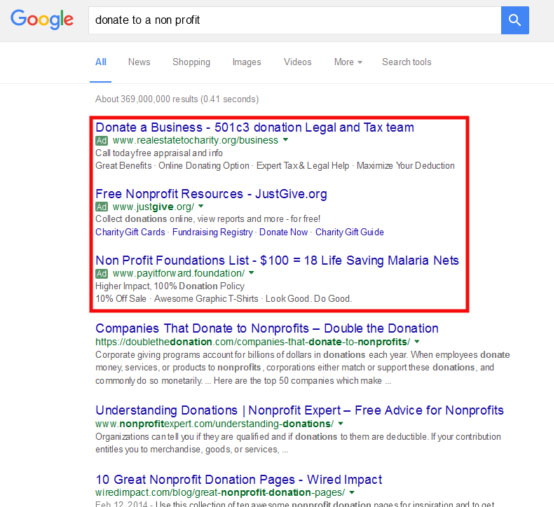The screenshot captures the results of a Google search query on a plain white background. At the top left corner, there is a light gray banner featuring the Google logo next to a search bar. Within the search bar, there is a magnifying glass icon encased in a blue square. The search query entered is "donate to a non-profit."

Below the search bar, a navigation tab is visible, offering options such as "All," "News," "Shopping," "Images," "Videos," "More," and search tools. The "All" option is highlighted in blue and underlined. The search results indicate approximately 369 million results, retrieved in 0.41 seconds.

The search results display a list of websites, each with a blue title link, a green font URL, and a gray description. Notably, the first three results are marked with small green boxes labeled "Ad," indicating that they are advertisements. These ads are enclosed in a red rectangle for emphasis. The urls and titles are as follows:

1. **Donate a Business - 501(c)(3) Donation Legal and Tax Team**
   
2. **Free Nonprofit Resources - JustGift.org**

3. **Nonprofit Foundations List - $100 Equals 18 Life-saving Malaria Nets**

The bottom three results do not have the "Ad" label, denoting they are organic search results.